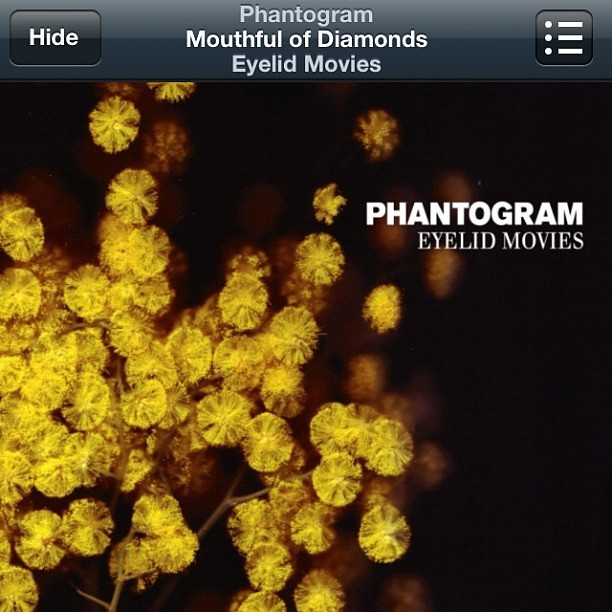The image appears to be an album cover with a primarily black background. The bottom left corner is adorned with approximately 30 tiny, golden star-shaped dandelions, attached to thin twigs. These resemble dandelions but are set on wooden stems, giving them a glittery appearance. At the top of the image, there's white text that reads, "Phantogram, Mouthful of Diamonds" on the first line, and "Eyelid Movies" on the second line. The text indicates that this might be a screenshot from a cell phone, as evident from a height button on the top left and a menu button on the top right.